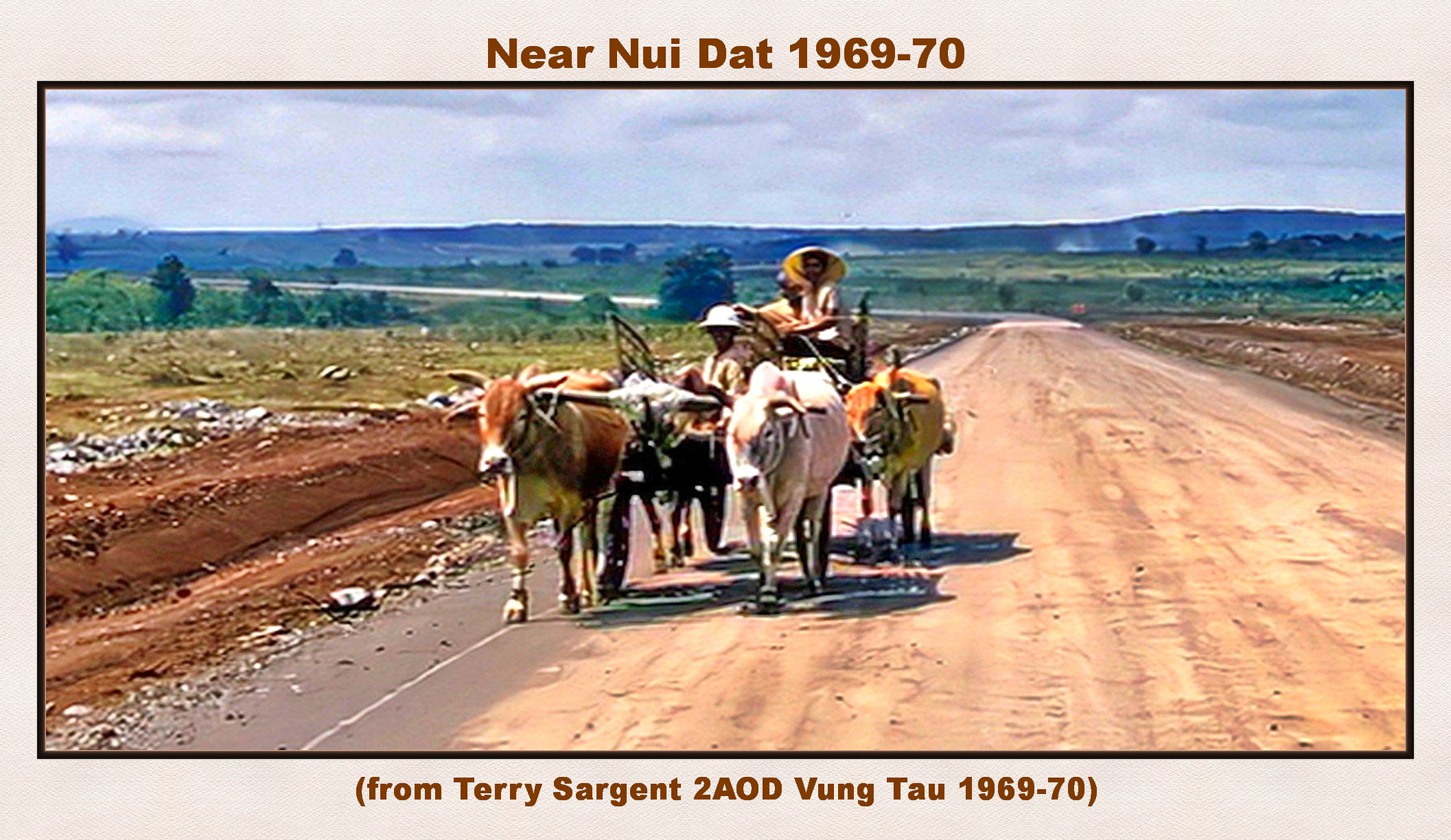An old, sepia-toned photograph encased in a light tan border captures a rural scene near Nui Dat from 1969-70. The top of the border reads "Near Nui Dat 1969-70" in brown text, while the bottom states "(From Terry Sergeant to AOD Vung Tau 1969-70)" in parentheses. The picture features a long dirt road meandering through expansive, sparse grasslands dotted with small trees. There is dirt and rocks on either side of the road, which curves to the left in the distance. The horizon is marked by low hills or a small mountain and a cloudy sky. At the forefront, a man donning a pointed hat with a wide brim is seen fussing with a team of four oxen, indicating their near exhaustion. The oxen are harnessed to a cart or carriage, with additional figures barely visible amidst the livestock. The scene depicted is reminiscent of the rural Vietnamese countryside during that era.